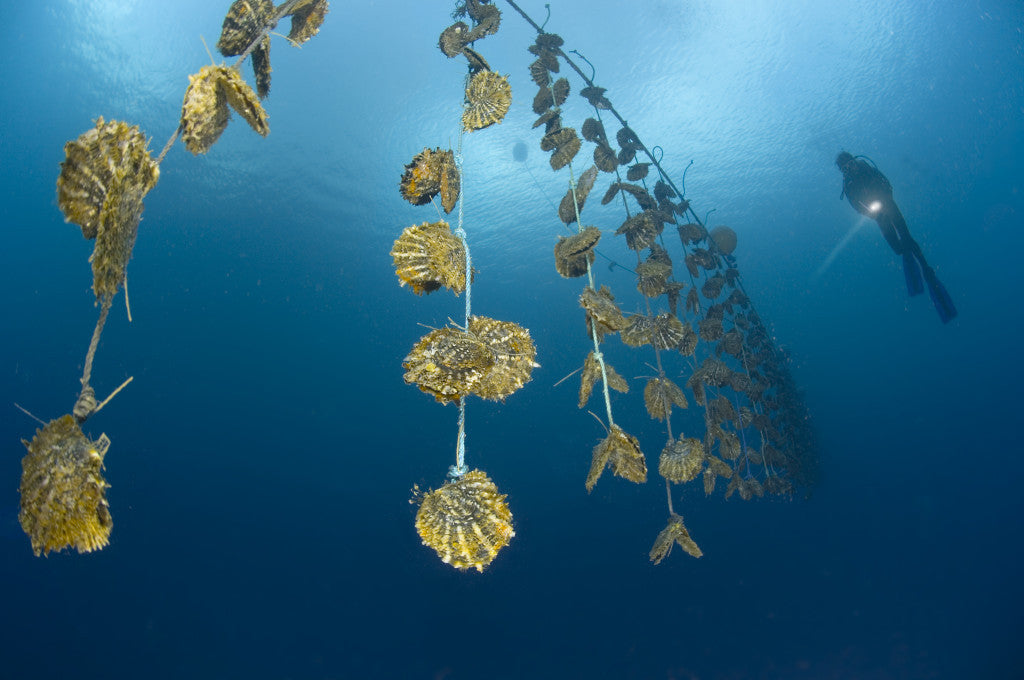In this underwater photograph, we observe a scuba diver silhouetted against the sunlight filtering from the surface, positioned in the background on the right-hand side. The diver is equipped with long swim fins, a wetsuit, and scuba gear, and holds a flashlight that casts a beam through the deep blue water. Suspended from a metal rod near the surface and extending downwards is a string or rope adorned with numerous algae- and moss-covered clam shells. These shells hang densely along the length of the rope, forming a striking vertical column that stretches far into the background, suggesting an underwater nursery or aquaculture setup. The scene captures the diver intently inspecting this marine growth, which adds to the image's depth and intrigue.